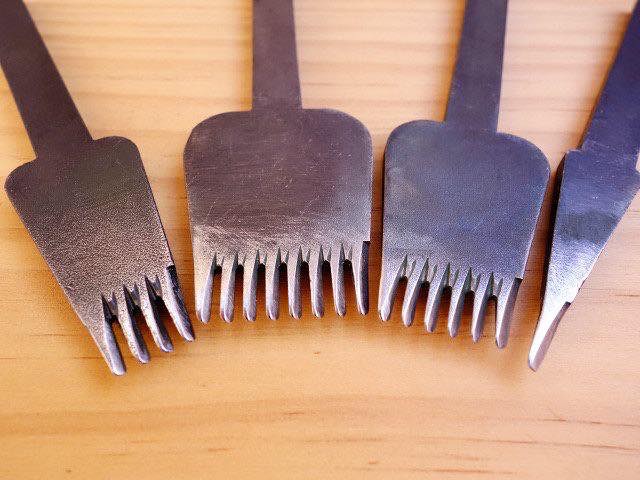This is a color photograph featuring four heavy metallic tools, possibly made of pewter, laid out on a light brown wooden surface. These tools appear to be specialized woodworking chisels or kitchen utensils with a distinctive fork-like design. Each tool varies in size and the number of prongs it has. From left to right, the first tool has four thick, short prongs, the second one has eight, the third has six, and the fourth tool is notable for having a single, sharp, triangular point. The tools are arranged in a slightly arched formation, with one tool lying on its side. Light reflects softly off their grayish-purple, metal bodies, accentuating their sturdy and heavy appearance.